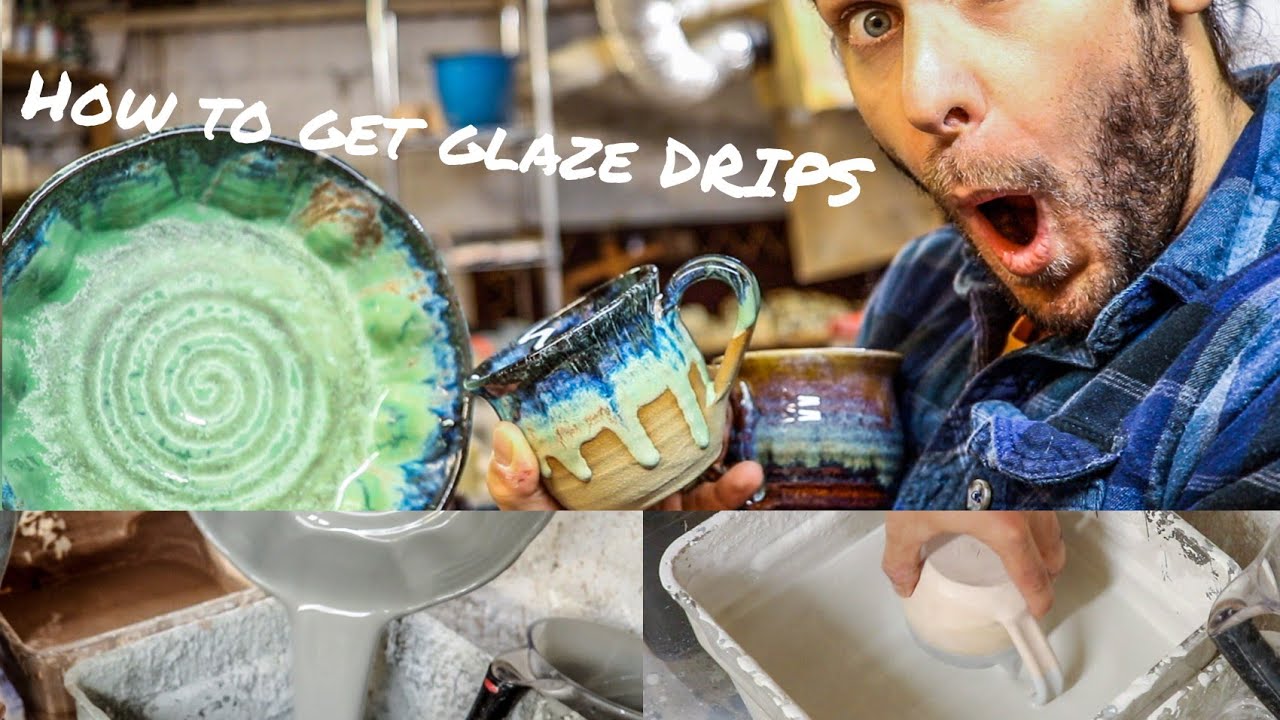The image is a collage comprising three photographs, prominently featuring a man in a blue and white plaid flannel shirt with a bit of a rough beard and light-colored eyes, displaying a shocked expression. He is holding two mugs and a small plate, all exhibiting colorful glaze drips. The overall composition seems designed for a YouTube thumbnail or article header for a DIY or ceramic art forum, emphasizing the process of achieving glaze drips on pottery. The man, captured from the nose down, is positioned on the right of the topmost, larger section of the collage, which spans the entire width and is labeled with white text reading "How to get glaze drips." The background suggests a warehouse or ceramic studio.

Below this top section are two smaller, closely cropped images. The left image shows a plate being dipped into a glaze, while the right image depicts a hand submerging a mug into a white bucket of glaze. These supplementary photos highlight the practical steps in the glazing process, reinforcing the instructional nature of the overall image.